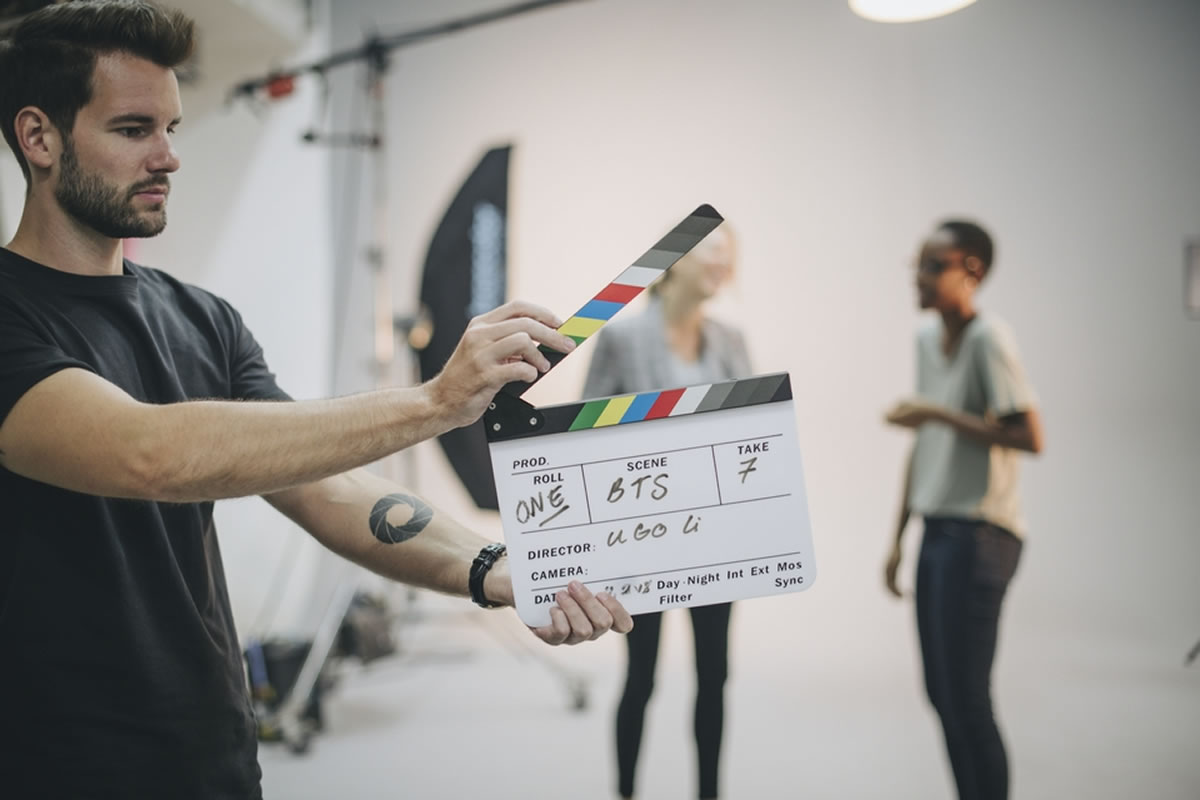The image captures a movie set scene, dominated by a young man, likely in his late 20s, holding a clapboard prominently. The man has a scruffy beard, brown hair, and a tattoo on his forearm, which appears to be tribal. Dressed in a black t-shirt, he is standing on the left side of the image, holding the clapboard aloft with both arms extended. The clapboard is colorful, with sections in green, yellow, blue, red, white, and gray. It displays handwritten details: "Roll: 1," "Scene: BTS," "Take: 7," "Director: Yugo Lee," alongside other partially obscured marks, including the date. 

In the blurry background, two figures are visible on the right side. One appears to be a thin Caucasian woman with black leggings and a gray jacket, leaning her head to the left and laughing. The second person could be either an African-American woman or a skinny man with short Afro hair and glasses, dressed in black jeans and a gray t-shirt. This person stands with their left arm bent and hand in front of their chest, engaging in conversation with the other individual. The setting is predominantly white, featuring a lighting rig on the left side and possibly a curtain, indicating an active film shoot.